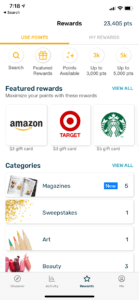This mobile screenshot showcases a rewards page. Despite being slightly blurry, the main elements are discernible. At the top, it features the word "Rewards" prominently displayed, with the current points, "2, 3, 4, 0, 6," indicated in dark blue text to the right. The page includes two tabs: "Use Points" on the left, which is highlighted and underlined in yellow, and "My Rewards" on the right. Beneath these tabs are five white buttons, each paired with a yellow icon, labeled as follows: "Search," "Preferred Rewards," "Points Available," "Up to 3,000 Points," and "Up to 5,000 Points." The "Featured Rewards" section is prominently displayed below these buttons, showing the logos of Amazon, Target, and Starbucks within white squares. A section for "Categories" is situated below the featured rewards.